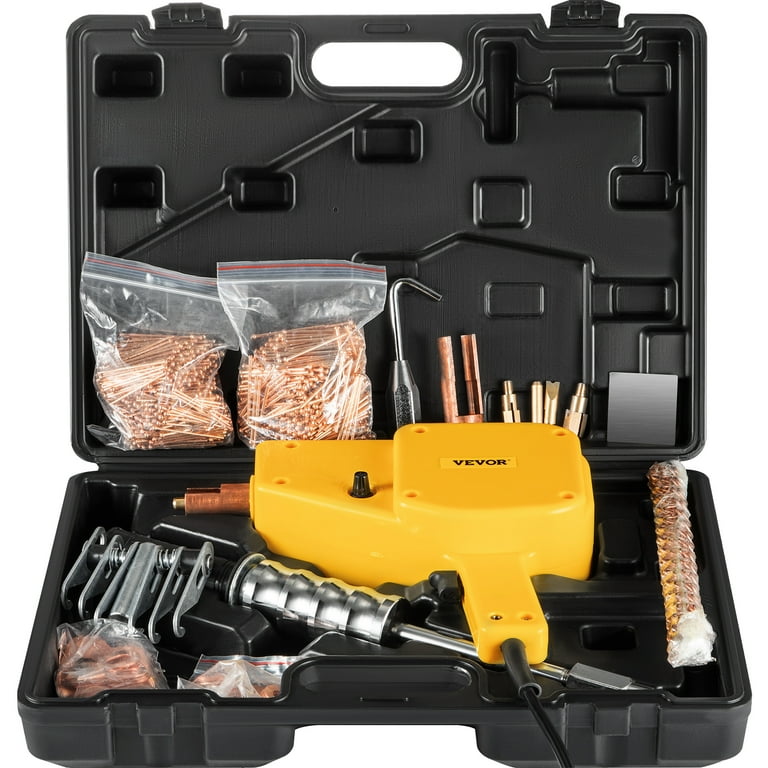This photograph showcases an open case containing a bright yellow riveting machine marked with the brand name "VEVOR" in black letters on its side. The sturdy black plastic case features custom-molded compartments designed to perfectly accommodate the tool and its accessories. The riveting machine itself, shaped like a nail gun with a copper-colored tip, includes a trigger and an extending cord.

Inside the case, there are various accessories neatly arranged in designated sections. This includes different riveting attachments and a long rod bit. On the right side, several bits are displayed, accompanied by a cleaning attachment and a small holder for the cord. On the left middle section, there are Ziploc bags filled with copper rivets, indicating the diverse functionality of the machine. The kit is designed to keep all components orderly and secure, making it a comprehensive set for riveting tasks.